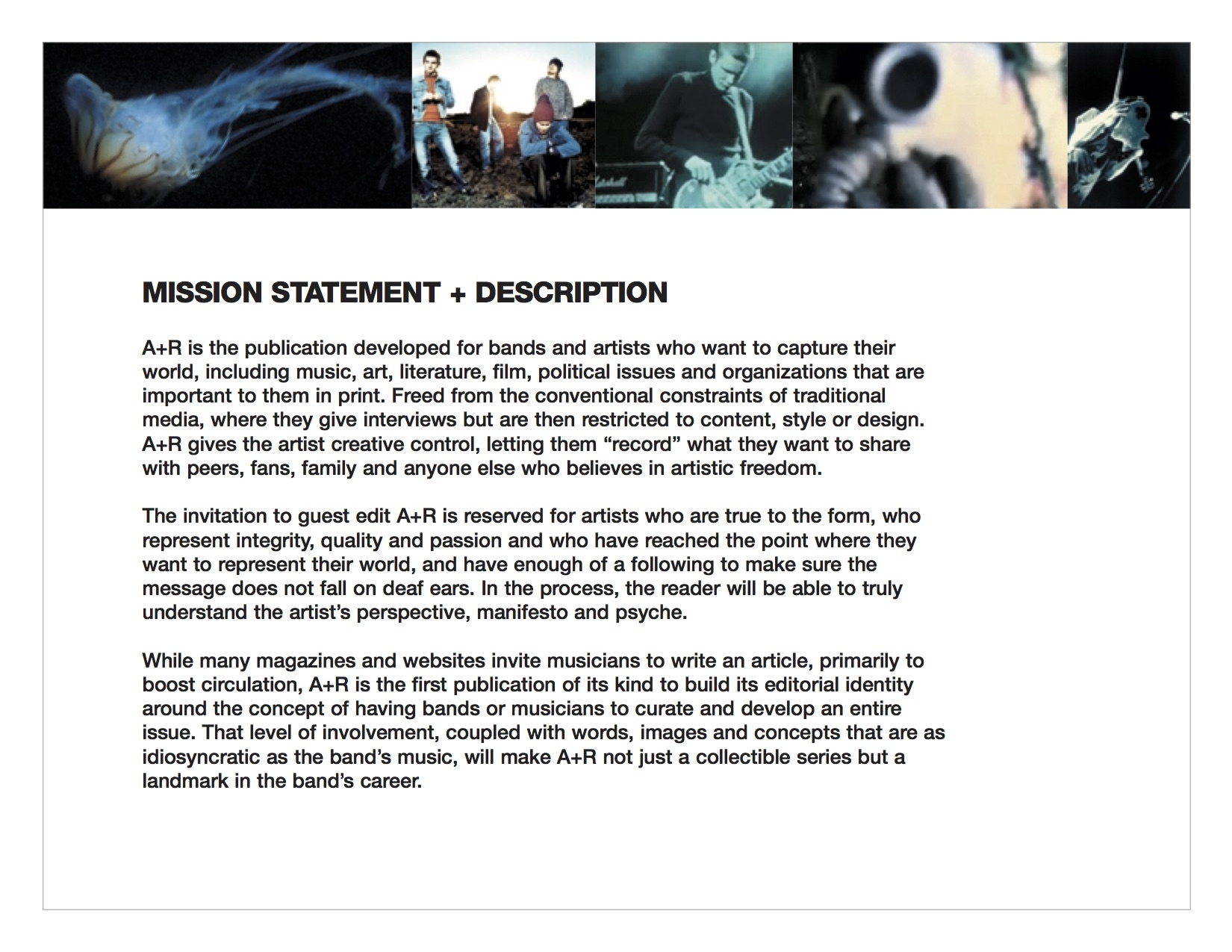The image showcases a mission statement for a publication called A&R, dedicated to bands and artists across various disciplines like music, arts, literature, film, and political issues. It includes a horizontal arrangement of five small square images across the top, set against a predominantly dark background with shades of black and blue. The first image is a jellyfish on a dark background, followed by a photo of four men in jeans standing in a field, then a man playing a guitar. The fourth image is blurry and indiscernible, while the fifth seems to show another person. Below these images, the mission statement text, printed in black on a white background, describes A&R as the first publication that allows artists complete editorial control to curate and develop entire issues. This idea is highlighted as a break from traditional media constraints, offering artists a platform for genuine self-expression. The publication aims to reflect the idiosyncratic nature of the bands’ music through their personally curated content, promising to be a landmark in their careers. The overall design features a mix of turquoise, red, orange, blue, gray, beige, and burgundy colors.